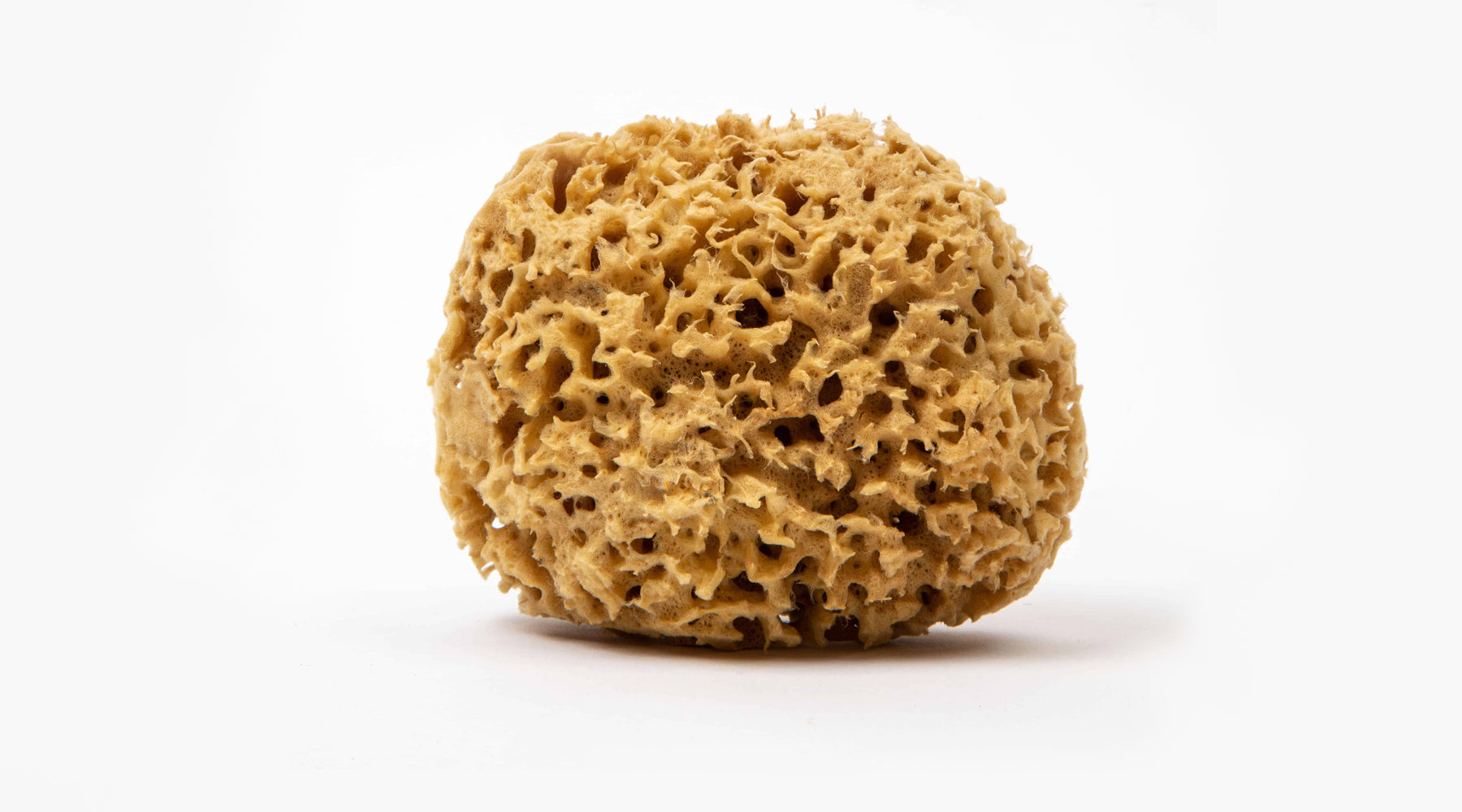The image showcases a close-up photograph of a natural sea sponge set against a clean, white background. The tan and brown round sea sponge is prominently placed at the center of the frame, casting a subtle shadow below it, indicating the lighting comes from above. The fine details of the sponge are highly visible, featuring cavernous holes and various intricate ridges and protrusions that are characteristic of a sea sponge. The texture appears complex and compact, suggesting it as freshly retrieved from the ocean. The sponge's natural fibers and small tentacle-like structures emanate a sense of life, as if this specimen once housed small marine creatures. Its relatively small size suggests it could comfortably fit in the palm of a hand, and might be used for personal care or display. The entire photograph focuses solely on highlighting the natural beauty and unique structure of the sea sponge.